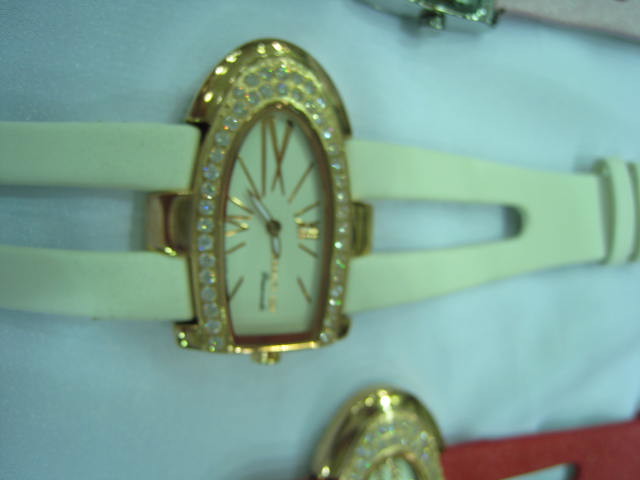In this image, three distinct watches are partially visible, each with unique features. At the top right corner, a silver watch with a light-colored band is faintly seen, showcasing a winding mechanism. The central focus of the image is a watch with a white band, adorned with a gold bezel that features Roman numerals. Surrounding the bezel are shimmering elements, potentially diamonds or another type of shiny stone, and the watch face has an unusual, elegant oval shape. At the bottom, barely noticeable, is another watch with a red band. It has a similar design to the central watch, including a comparable case and bezel decorated with clear, sparkling stones.